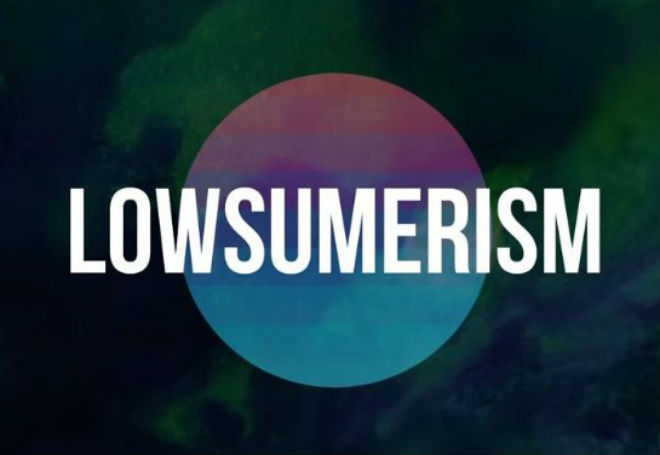In the center foreground of the image, bold white text spells out "Low Summerism." Directly behind the text lies a large, silvery-white sphere that gradually transitions from teal at the bottom to purple at the top. The sphere is set against a dark, textured background composed of various dark hues, including smoky green, rusty black, and deep blue. The background colors blend and fade into each other with some areas appearing more granular and blurry, particularly the irregular patches of dark green and black. The darkest sections of the image are located in the upper left and bottom left corners, which are nearly solid black, while the bottom right corner features a mix of black, dark green, and dark blue shades. The upper right corner has a mix of dark green and black, creating a contrast against the vivid sphere. Overall, the image has an illustrative quality, resembling a stylized drawing more than a photograph, and its dimensions are wider than it is tall. The simplified composition suggests it could be an advertisement for a show or a music festival.